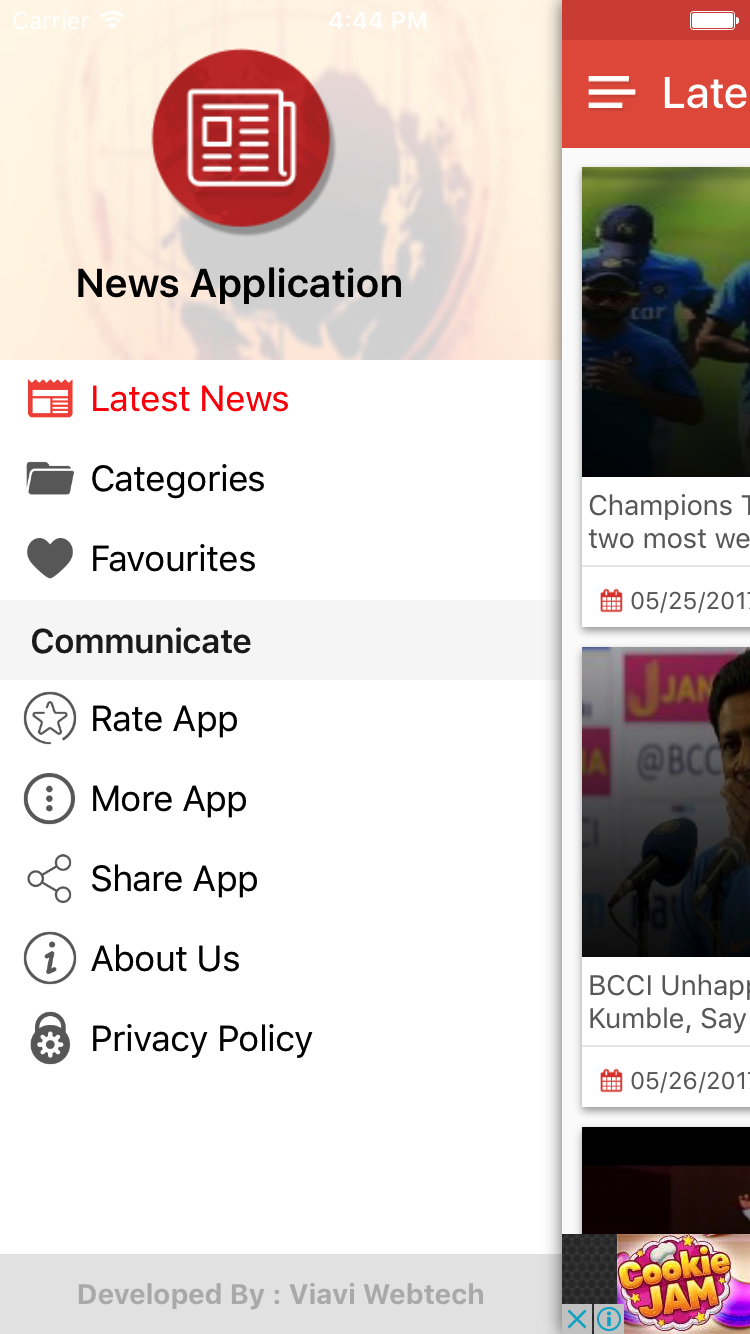**Detailed Caption of a Tall Rectangular Image**

This image is a tall, portrait-oriented rectangle, akin to the shape of a cell phone screen. The visible part of the image primarily shows the left panel of what appears to be a two-panel online computer webpage, with about 80% of the left panel displayed and the right panel cut off.

**Left Panel Description:**

- **Backgrounds and Layout:**
  - The upper third of the left panel features a light beige background.
  - The bottom 10% of the panel has a gray background.
  - The middle section, taking up the majority of the panel, has a white background.

- **Content in Upper Beige Background:**
  - Centered in the upper beige section is a red circle with a simplistic white newspaper icon, displaying lines to indicate text and a small square to signify an image.
  - Below the red circle, in black text, it reads "News Application."

- **Content in White Background:**
  - Nine different words/phrases are aligned to the left, each with varying icons.
  - The first three entries consist of black icons:
    - "Latest News" (red icon resembling a folded broadsheet newspaper)
    - "Categories" (black icon of an open folder)
    - "Favourites" (British spelling with a dark gray filled heart icon)
  - Below these, on a light gray background, the word "Communicate" is displayed without an accompanying icon.
  - The next five entries, each featuring gray icons, include:
    - "Rate App" (circle with a star icon)
    - "More App" (circle with three vertical dots icon)
    - "Share App" (icon resembling an atom with three circles connected in a triangle shape)
    - "About Us" (circle with a lowercase "i" information icon)
    - "Privacy Policy" (lock icon)

**Right Panel Description:**

- The right side of the image is partially visible, revealing fragments of three pictures or videos:
  - The top portion shows a red banner with partially legible white text reading "Late...". A white battery icon in the upper-right corner indicates full power.
  - Below are glimpses of what appears to be a sporting event. Participants are wearing blue caps, possibly suggesting a cricket match. Fragmented text reads "Champions" and "To Most," alongside a red calendar icon and the date "05/25/2011."
  - The middle image shows about 90% of a person at a microphone.
  - The bottom portion shows an image related to "Cookie Jam."

- In the bottom left corner, inside a light gray section, darker gray text states: "Developed by: via the WebTech."

Thus, the image provides a detailed glimpse of an online news application interface, replete with various navigational options and partially visible multimedia content.